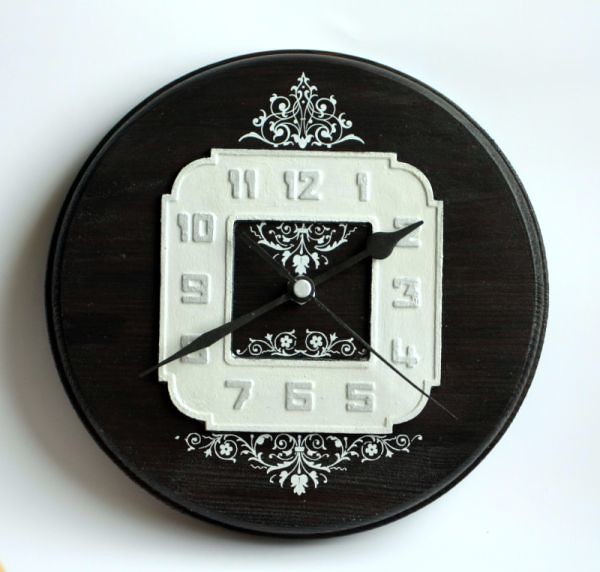The image showcases an intricately designed clock made of very dark wood, almost black in appearance. The clock features a white face adorned with black hands, making it somewhat challenging to discern the exact time, which reads approximately 2:40. At both the top and bottom of the clock, there are ornate white floral designs that add a touch of elegance. The background of the photo is white, and a shadow is cast to the left, adding depth to the composition. Despite its craftsmanship, the clock may not appeal to everyone's taste, as the observer describes it as fairly unattractive.